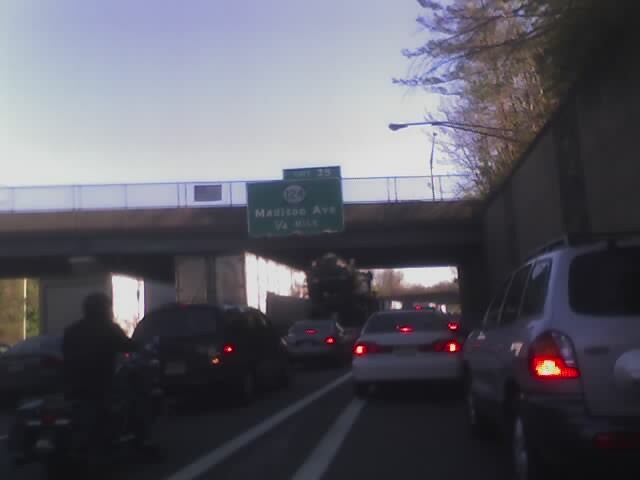In this low-light, blurry photograph, we see a road stretching into the distance under a greyish, cloudless sky. The image is framed by trees in the upper right-hand corner and a bridge crossing over the road. The bridge features a green sign with white lettering, though the text is too dark and blurry to decipher. Several vehicles populate the road ahead, including both greyish or white cars and darker vehicles on the left. Their red taillights glow against the dim backdrop, with each vehicle emitting a distinct pair of lights. Near the back of the image, there seems to be a faint outline of a person, possibly on a motorbike, though it's challenging to discern. In the very left-hand corner near the bridge, some illuminated foliage suggests the presence of evening sunlight filtering through. White lines on the road are faintly visible, guiding the flow of traffic.